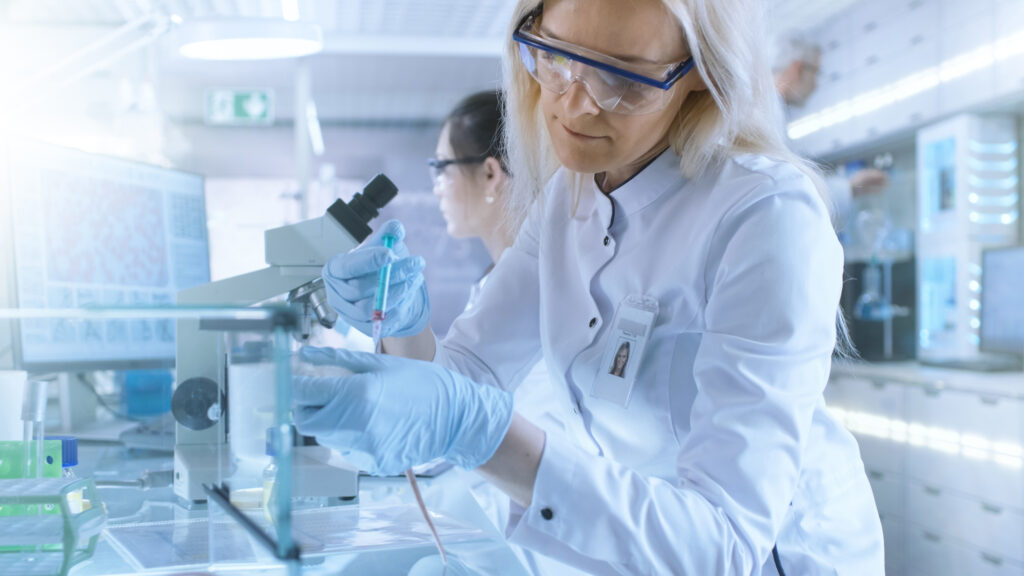This stock image captures a pristine, bright white laboratory filled with high-tech equipment and busy scientists. On the left side, white drawers line the wall, topped by computer equipment encased in illuminated white units with neon blue panels. Central to the scene is a reflective white table cluttered with lab tools, including a yellowish-white microscope with black dials and eyepieces.

In the foreground stands a prominent female scientist. She has long blonde hair, wears a white lab coat with a name tag featuring her picture hanging on the right side of her chest, and protective goggles with a blue strip across the top. Her hands, clad in blue latex gloves, dexterously hold a needle filled with bright blue liquid in her right hand and a Petri dish in her left.

In the background, another scientist with brown hair tied back into a ponytail, equally equipped with safety goggles, is intently focused on a large computer screen displaying complex blue diagrams. Beside her are a pair of binoculars, further emphasizing the meticulous nature of the lab work being conducted. The overall ambience is sterile and illuminated by strips of lights on the walls and ceiling, enhancing the lab's cleanliness and high-tech aura.